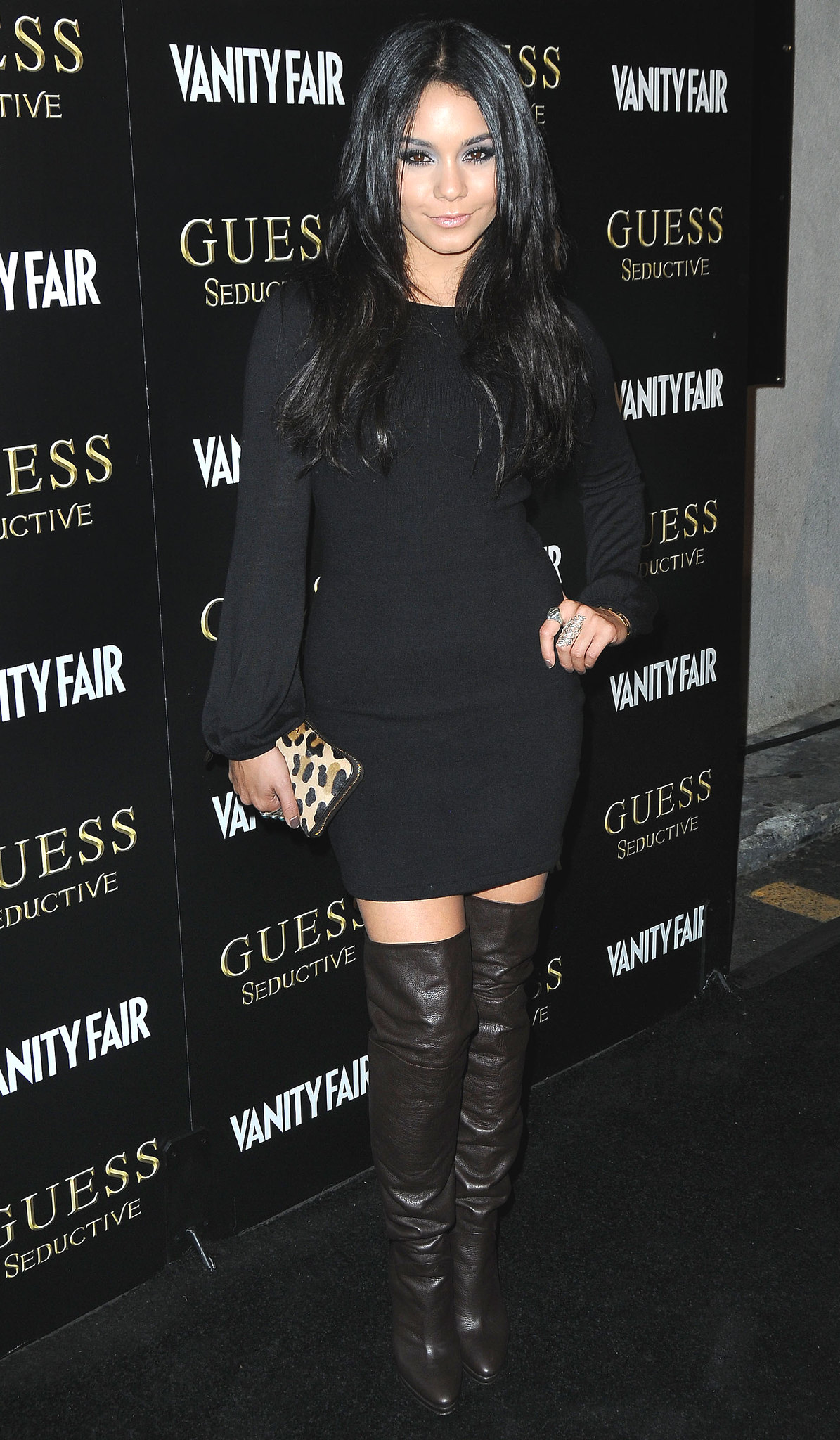In this striking digital photograph taken at a Vanity Fair event, actress Vanessa Hudgens stands poised and confidently facing the camera. She exudes elegance in a long-sleeve, short black dress paired with thigh-high black boots that appear to be crafted from leather. Her right hand elegantly holds a chic leopard print handbag, and she accessorizes with prominent silver rings, particularly noticeable on her left middle finger. The backdrop features an array of black signs that repeatedly display the words "Vanity Fair," "Guests," and "Seductive" against a plain white wall. The actress stands upon a plush black rug, completing the sophisticated ambiance. To the side, a yellow line marking is faintly visible in the distance, further adding to the detailed setting of the scene.